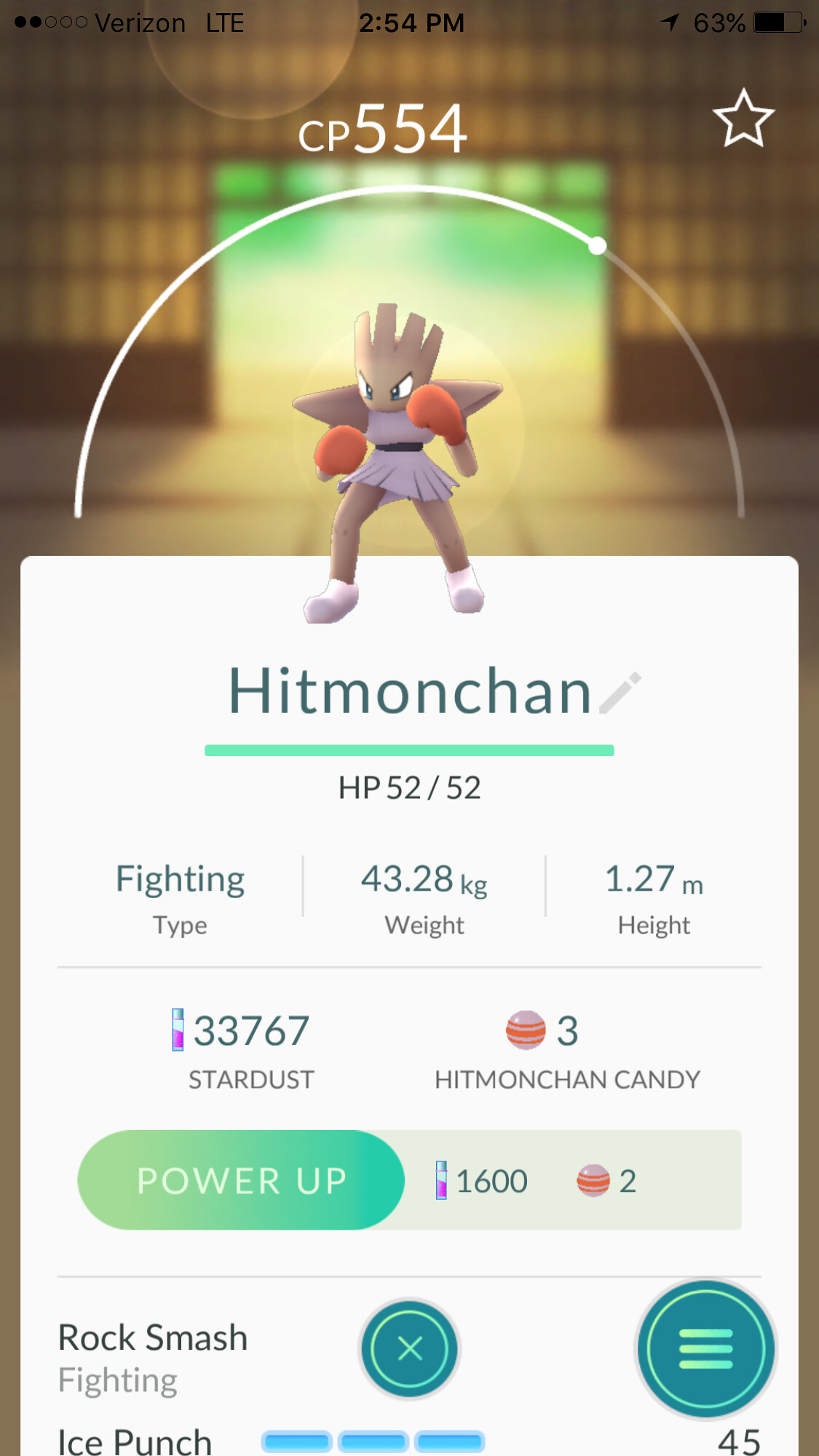The image depicts a screenshot from a Pokemon mobile game, featuring the character Hitmonchan in the center of the screen. Hitmonchan, a fighting-type Pokemon, is dressed in a purple dress with orange boxing gloves and white shoes. The character has spiky hair and large, angry cartoon eyes. The backdrop consists of a brown, door-like area. Above Hitmonchan's head is a semicircular progress bar with the label "CP554" and a star icon in the top right corner. The display shows detailed stats: HP is 52/52, weight is 43.28 kilograms, and height is 1.27 meters. Hitmonchan has accumulated 33767 Stardust and 3 Hitmonchan Candy. Available moves include Rock Smash (Fighting-type) and Ice Punch. On the left-hand corner, there is a button marked with an "X" and "45." The game information, such as the battery life of 63%, time stamp of 2:54 p.m., and Verizon LTE connection, is visible on the screen.